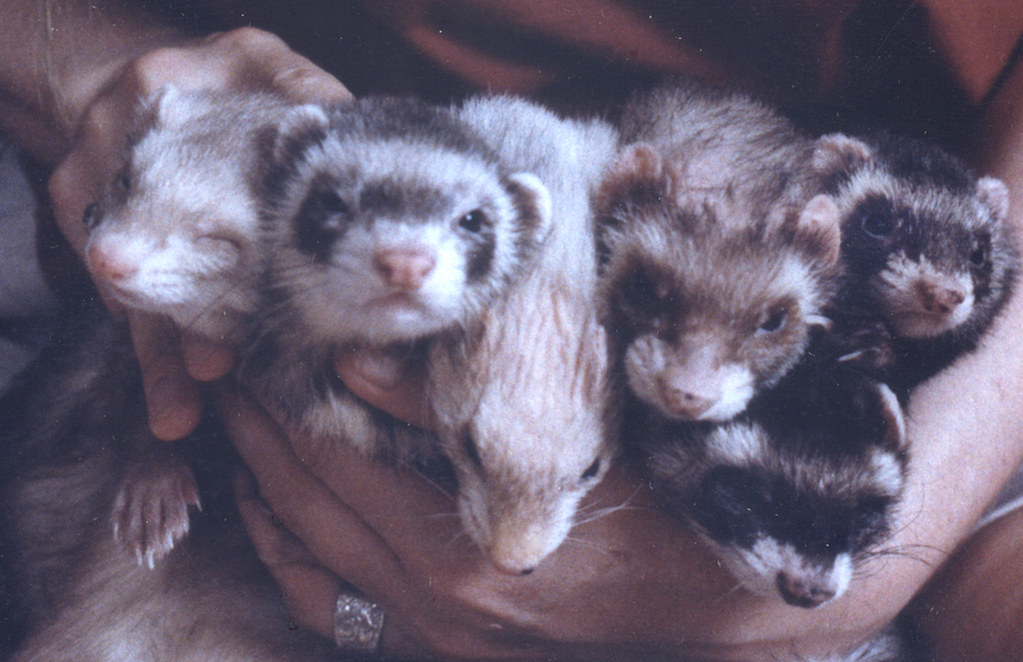In this detailed photograph, six ferrets are being carefully cradled by a person whose hands are the only visible parts of their body, other than the crimson-colored shirt they're wearing. The person appears to be of European descent and is likely male, wearing a silver wedding band on the hand supporting the ferrets from below. The ferrets are nestled closely together, fitting comfortably in the individual's two hands. All of the ferrets are looking directly at the camera, displaying their characteristic whiskers and pink noses. 

The coloration of the ferrets varies slightly, with two exhibiting a darker black hue, while the other four display different shades of gray, light brown, and beige. Specific details include a beige ferret with a notable white spot around its nose, typical of ferret markings. Additionally, their small, rodent-like appearance is accentuated by the visibility of their five-toed paws with needle-sharp nails. This captivating image puts the ferrets at the focal point, highlighting their unique features and the gentle care of the person holding them.